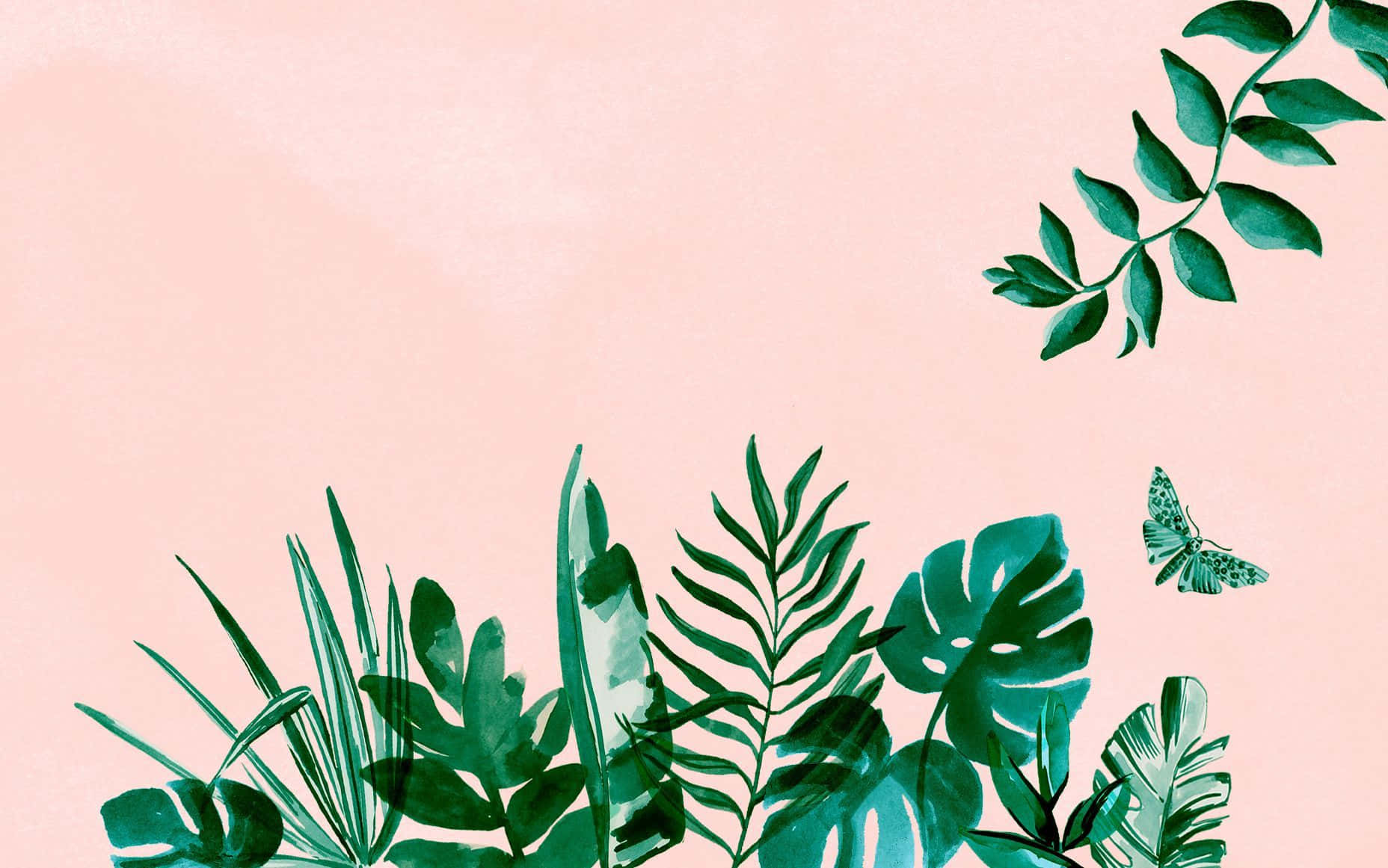This image depicts a richly detailed painting set against a peach-colored background. The composition features several green plants positioned at the bottom, displaying a variety of leaf shapes such as broad, narrow, conical, and needle-like, each contributing to a lush, textured scene. One prominent plant located in the top right corner extends a stem downwards, adorned with pairs of leaves on each side until it culminates in a single leaf at its tip. In the central part of the image, there is a striking green butterfly with black spots. Its body is oriented downward, while its antennae stretch upward. The butterfly's wings are splayed, giving the impression that it is gracefully flying toward the lower right of the picture. This vertical and upward interplay between the plants and the butterfly creates a dynamic visual balance in the artwork.